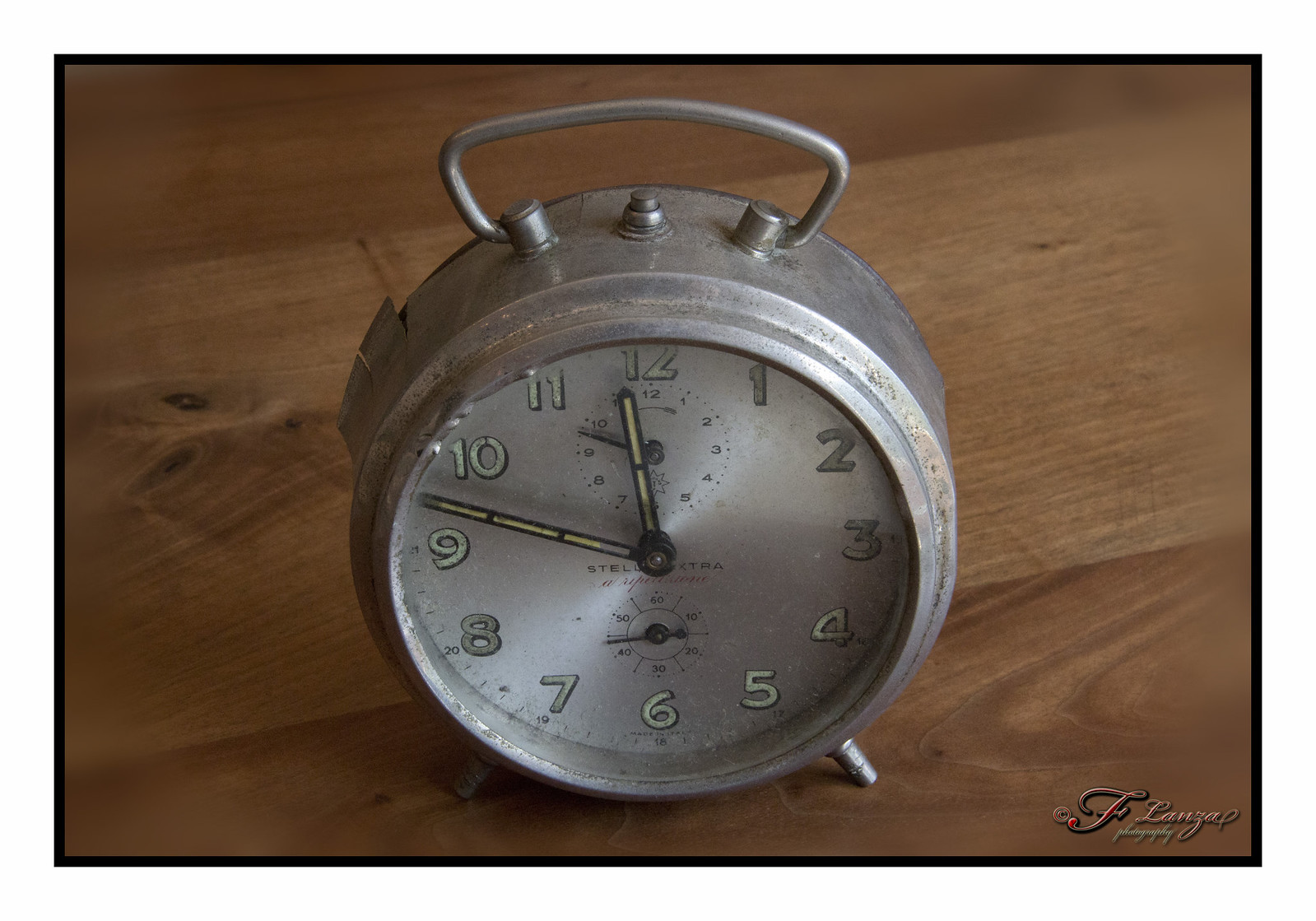The image captures an antique-style, silver-colored metal alarm clock prominently placed in the center on a richly grained wooden table. The clock features a slightly rusted and worn exterior, suggesting age and oxidation. It has a wire handle at the top, accompanied by three buttons, and four small legs at its base for stability. The clock face is silver with black hands accented by faded green, possibly once fluorescent, which might still glow in the dark. The numerals, matching in pale green, also seem designed to be luminous. At the top of the clock face, there is a small button, while at the bottom, additional dials likely serve as indicators for seconds or perhaps days of the week. The time displayed is just past quarter to twelve. In the bottom right corner of the photograph, there is a barely legible watermark, presumably indicating the photographer's name. The warm, textured wooden surface beneath the clock adds to the vintage aesthetic, emphasizing the clock's historic and well-used appearance.